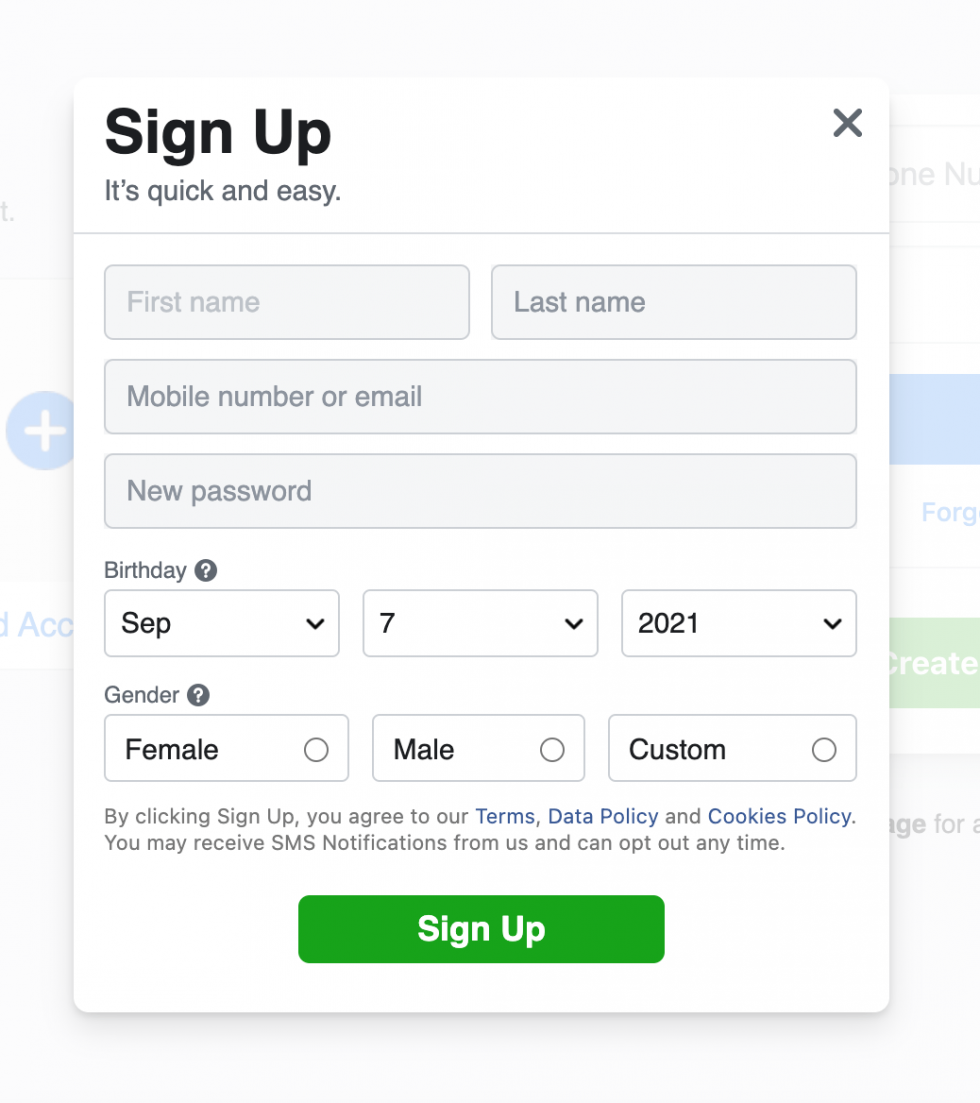The image depicts a sign-up form presented as a pop-up window, likely for a smartphone app but possibly on a computer. The background is grayed out, emphasizing the pop-up, which features a subtle drop shadow.

At the top of the pop-up, bold text reads "Sign Up, It's Quick and Easy" with a close ("X") button in the upper right corner. The form contains several entry fields: side-by-side fields for "First Name" and "Last Name," followed by a full-width field for "Mobile Number or Email." Below this, there is another full-width entry field for a "New Password."

Further down, the form asks for the user's "Birthday," with drop-down menus indicating that "September" has been chosen for the month, "7" for the day, and "2021" for the year—though this year is obviously incorrect. 

The next section is for "Gender," offering three options: "Female," "Male," and "Custom," with none of them selected. Beneath the gender options, smaller gray text indicates, "By clicking sign up, you agree to our Terms, Data Policy, and Cookies Policy. You may also receive SMS notifications from us, and you can opt out at any time."

A prominent green rectangular button at the bottom displays the text "Sign Up" in white. The overall appearance of the form is predominantly white, with not enough detail in the background to describe it further.